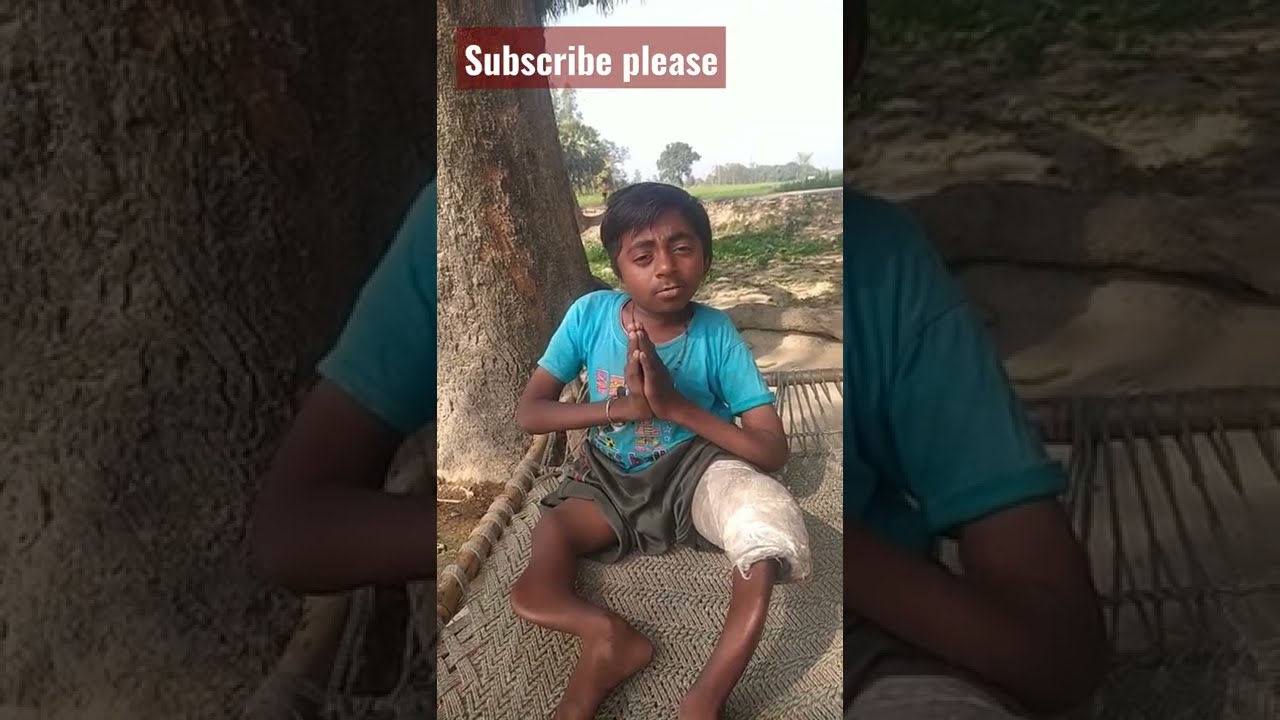The photograph, likely taken on a phone, features a young boy with dark brown skin, possibly of Indian descent. Positioned centrally, the photo is accompanied by enlarged, darker duplicates on either side. The boy, who has a disability affecting his legs, is sitting on a beige hammock next to a large tree with a vast sandy and grassy field in the background. He has short, straight black hair that reaches his ears. His hands are clasped together in a prayer pose, and he is wearing a light blue t-shirt and olive-green or gray baggy shorts. His legs are notably deformed; the left leg appears particularly misshapen and the right leg has a white cast from the upper thigh to the knee. At the top of the image, a red rectangular banner with white text reads, "subscribe please." The overall composition gives a poignant insight into the boy's condition and surroundings.